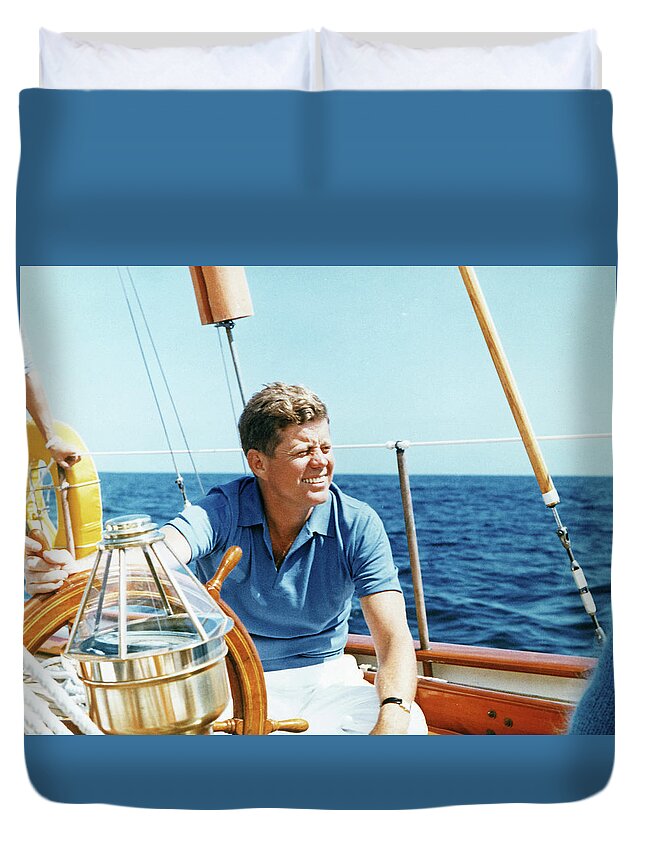In this detailed color photograph, John F. Kennedy is seen enjoying a day on the water aboard his sailboat. The former president is seated near the wooden steering wheel, which he holds with his right hand, steering the boat. His attire includes a blue polo shirt and white pants. Kennedy, smiling broadly, gazes off to the right, with his short hair catching the sunlight. His left arm is propped on his knee in a relaxed posture. The boat itself features a lot of wood paneling, with a metal riser wrapped in white rope serving as a railing. Behind him, there are steel pulleys attached to the sail supports, and ropes extending towards the mast. The background reveals a bright blue sky and the deep blue ocean surrounding the boat. A clear jug and what appears to be a golden lantern are also on the boat, adding to the nautical atmosphere. The image is presented in landscape orientation and is superimposed over a color illustration of a bed, with the photograph acting as a blanket over the midsection. The illustration includes a blue blanket cover and white pillows extending from the top edge, blending photographic realism with illustrative elements.